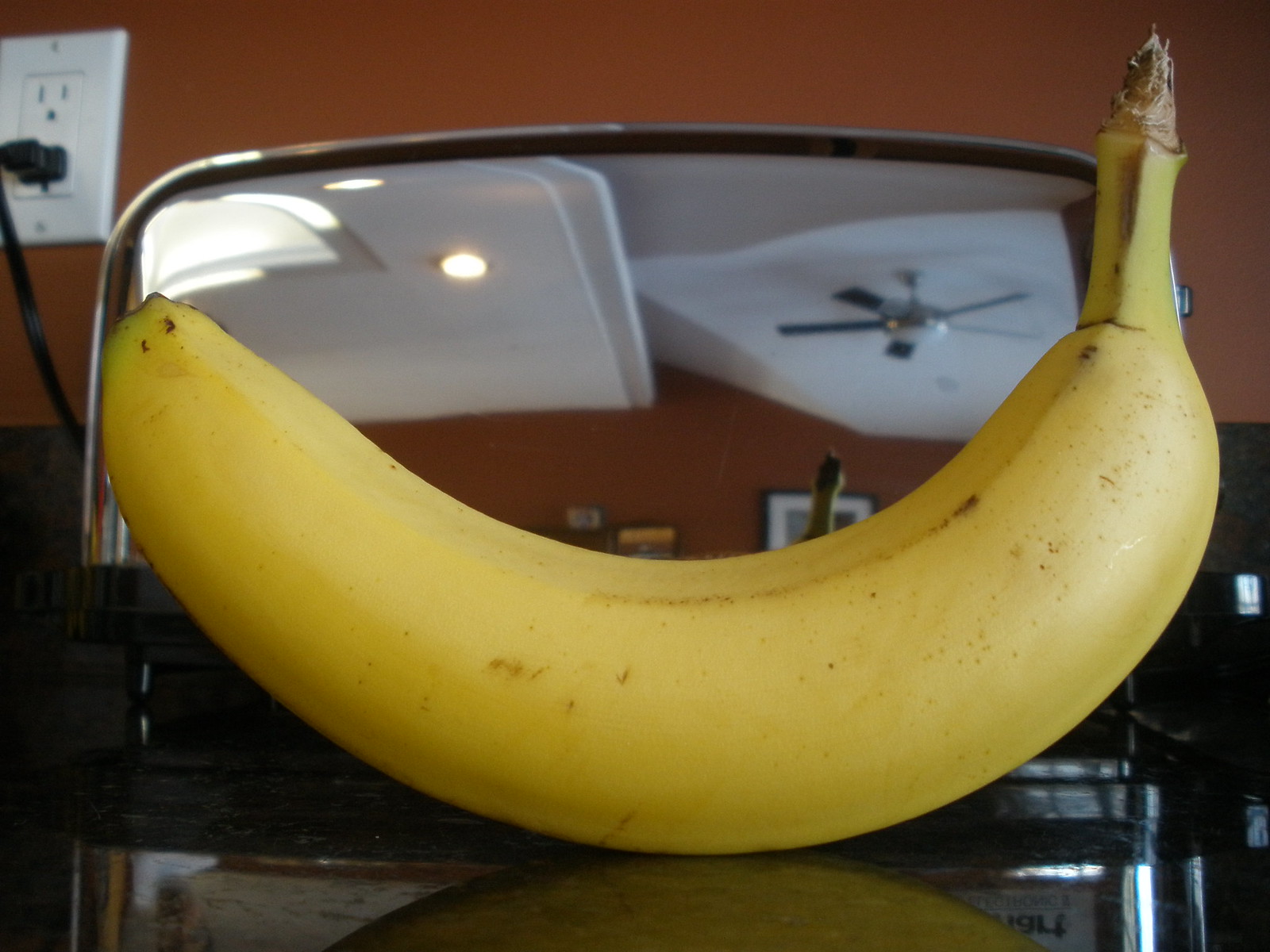In this captivating image, a perfectly smooth, vibrant yellow banana is prominently displayed on a reflective silver metal surface. The banana, exhibiting a nearly flawless exterior, features a brown pointed stem at the top and a few subtle brown speckles on its right side, adding a touch of natural texture. Behind the banana, a vivid red wall enhances the contrast and brings out the fruit's vivid hue. 

A white electrical outlet is visible in the upper left corner, with a black cable plugged into the bottom socket, contributing to the everyday setting. The reflective surface beneath the banana not only mirrors the fruit but also other elements of the room, revealing details like a white ceiling, a couple of lights, and a silver ceiling fan, slightly distorted due to the curvature of the surface. 

In this mirrored backdrop, the ceiling and the wall behind the banana are also visible. The opposing wall, sharing the same rich reddish-orange hue, features part of a black-framed painting or similar object, adding depth to the scene. The reflection on the silver surface captures the top of the banana, including its brown stem, merging seamlessly with the overall composition and providing a fascinating interplay of real and reflected imagery.